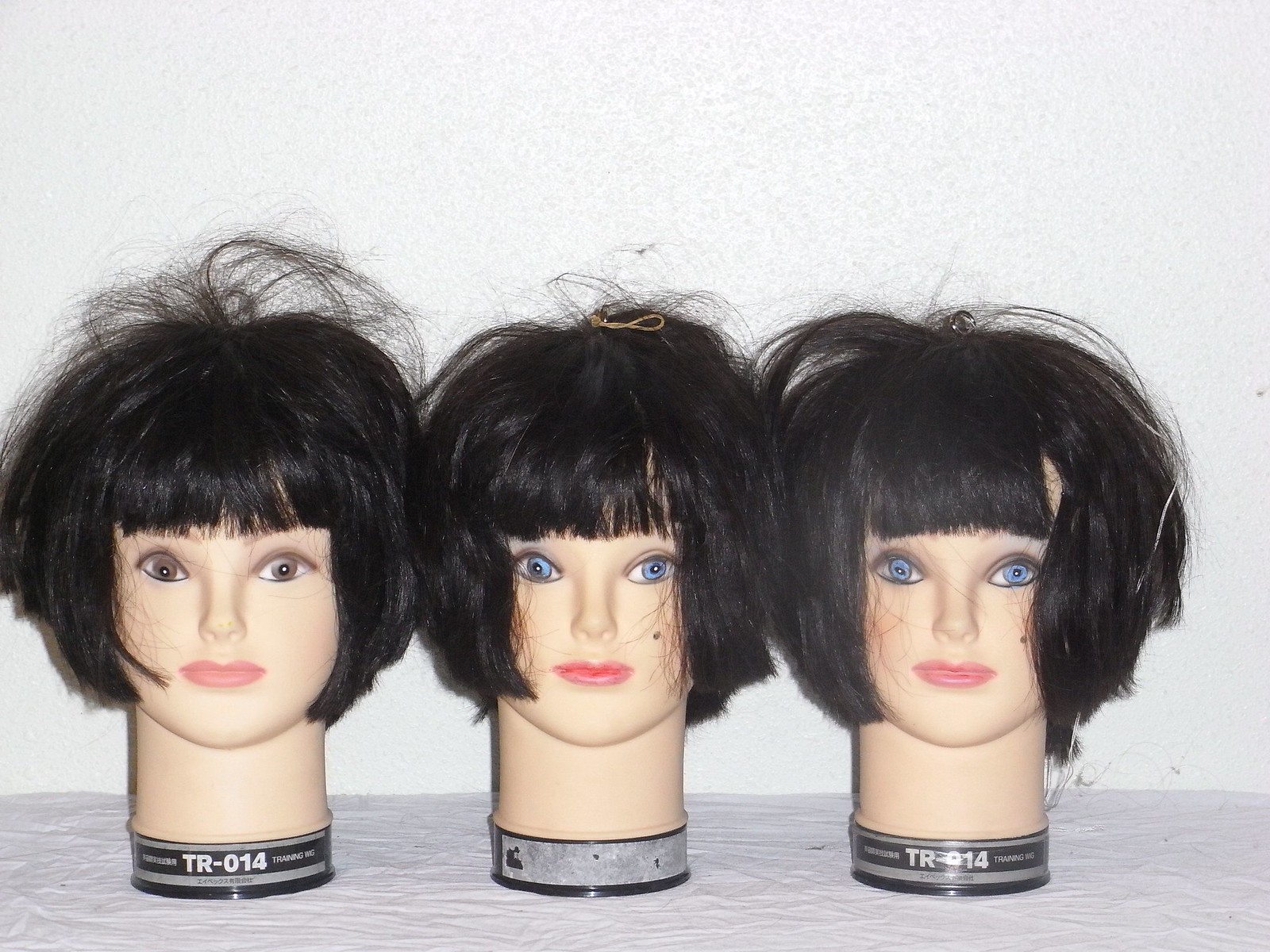This image features three Caucasian mannequin heads lined up side by side on a white textured counter, set against a white popcorn-textured wall. Each mannequin sports a short brunette wig with bangs. The mannequins display slight variations in hairstyle despite the overall similarity. The mannequin on the left has brown eyes and pink lips, with a short, layered haircut that appears unkempt, with several stray hairs. It has the code "TR-014" around its neck. The middle mannequin has bright blue eyes and a bushier, straight hairstyle, while the right mannequin, which has the same eye color and head type, presents a less full, more straightened version of the same haircut, also featuring flyaway hairs. Notably, two mannequins have hair ties in their hair, and all bear styling similarities typical of those used in hair salon schools for practice.